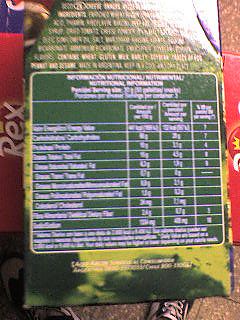The photo captures a downward view of a partially blurry, dark green menu or nutritional label laying on a red table. The table features the word "Rex" both on the left and right edges. The menu itself has white text at the top, a centrally located darker green square with white writing arranged in columns that suggests nutritional information like ingredients and caloric content, and potentially company information at the bottom in smaller white text. Despite the blurriness, identifiable ingredients include wheat flour, wheat gluten, barley, and tomato. Partially visible at the bottom of the image are a pair of black lace-up shoes, resembling Vans, standing on a brown and white tiled floor.